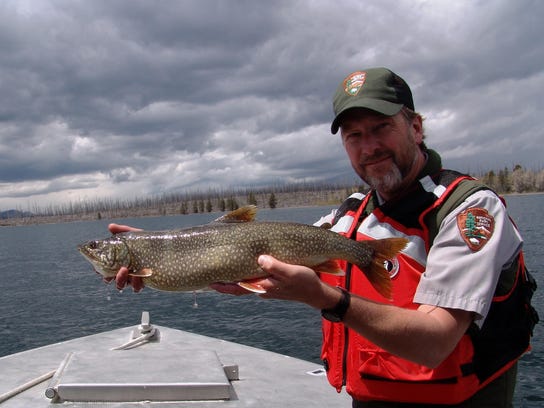In the photograph, a man stands on a silver boat against a backdrop of a cloudy, gray sky that hints at an impending storm. The boat cuts off at his waist, leaving him visible from the torso up. The man proudly holds an elongated, green fish with yellow spots and a white underbelly, its tan-colored fins contrasting sharply with its dark body. He has his left hand positioned under the fish and his right hand gripping its head, extending it outwards.

His attire includes a bulky, puffy, orange life vest with a zipper down the front, white stripes, and black shoulders. Underneath, he wears a gray short-sleeved shirt decorated with a logo of a governmental park agency on the visible left sleeve. A similar logo adorns his green baseball cap. The man's face, topped with a gray and brown beard, faces straight forward, displaying a slight smile of accomplishment.

The setting around him features a body of water leading to a shore with sparse, mostly dead trees and a few live ones peeking into the center of the image. The overall scene captures the man's triumphant moment, possibly having just caught the fish, beneath the darkening sky on the open water.